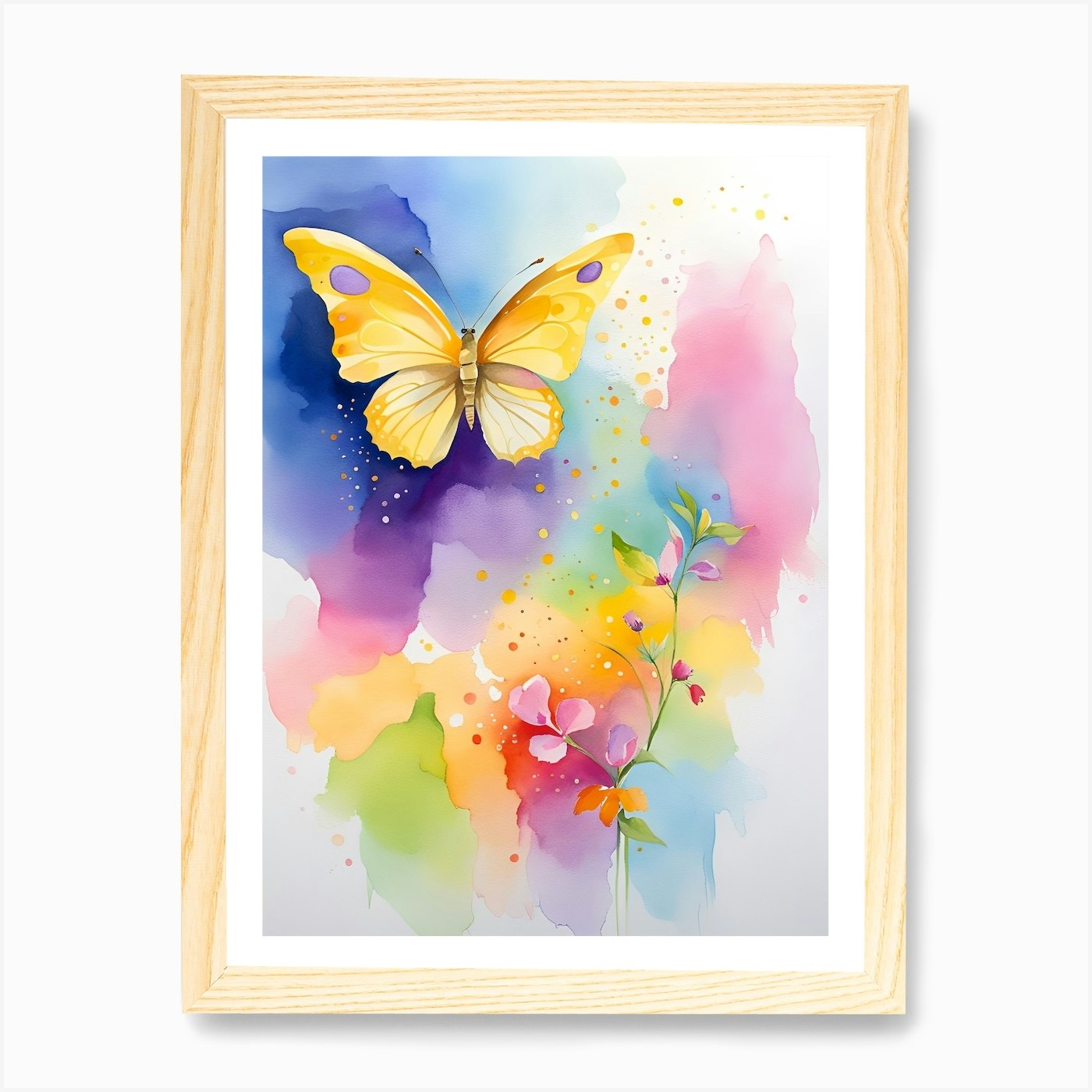The image showcases a digital preview of an art piece set against a white background, encased in a light birch wood frame with an additional white inner frame. The painting itself is an abstract watercolor composition featuring a splashed and blended backdrop of vibrant and muted hues including deep purples, dark and light blues, greens, yellows, pinks, reds, and turquoises. Centered within this colorful tapestry is a multi-colored plant emerging from the lower half, adorned with pink petals, budding flowers, and green stems. Toward the top right of the painting, a striking yellow butterfly with purple dots on its wings hovers against the dark bluish-purple background, with scattered specks of paint creating a subtle sparkle effect that interlaces between the butterfly and the plant. The bright colors and detailed elements of the plant and butterfly stand out vividly against the harmonious and fluid watercolor backdrop, making it a captivating and dynamic piece of art.